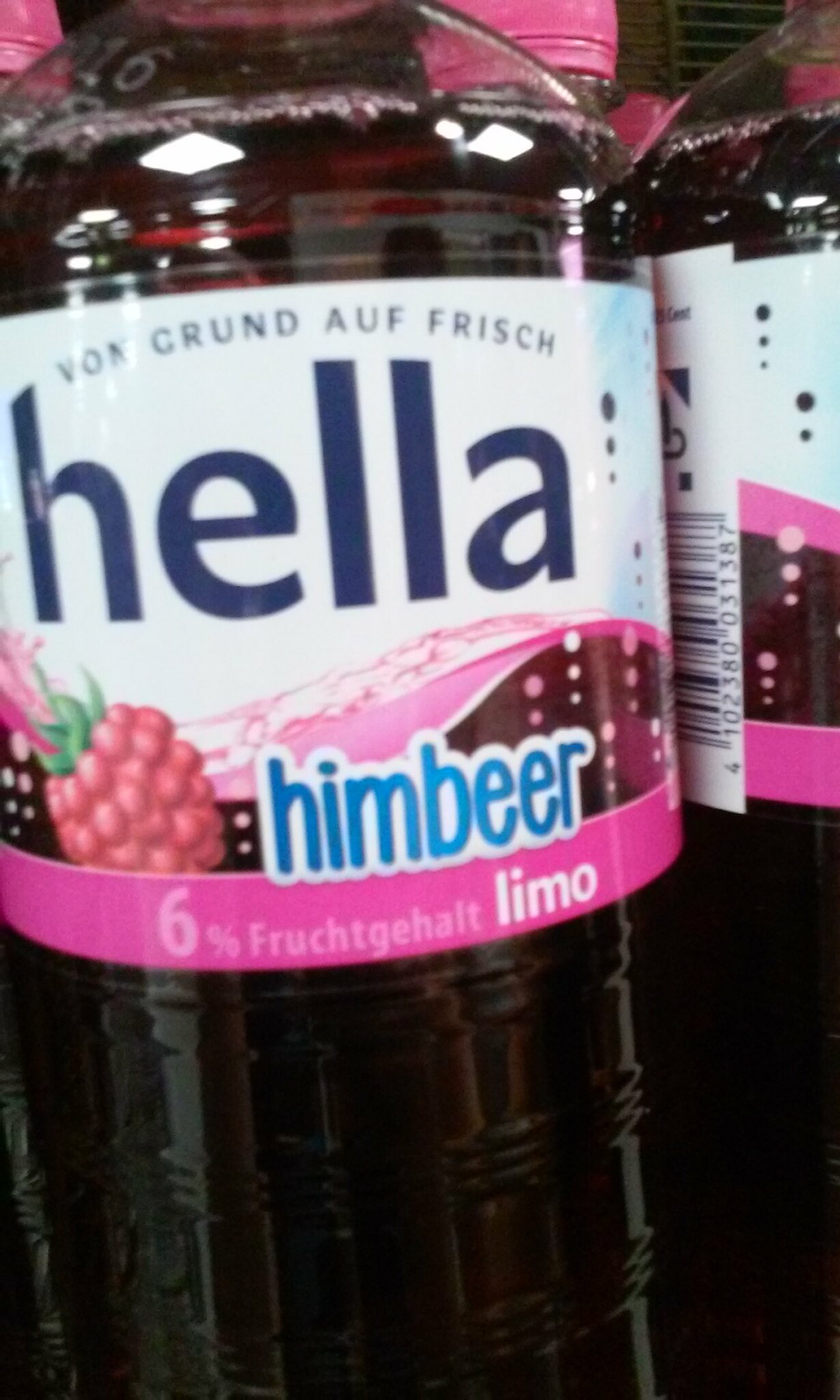This image shows a close-up of several clear plastic bottles filled with a dark maroon or deep purple juice, predominantly featuring one bottle at the forefront. The primary bottle sports a detailed label that is predominantly white with a pink border at the bottom. The label prominently features the word "HELLA" in large blue text, a fruit motif that appears to be raspberries, and additional text in blue reading "HIMBEER," indicating raspberry flavor. The label also includes a section with a pink background reading "6% Fruchtengraupt Limo" and imagery of juice flowing amidst the fruit illustrations. Additionally, the bottle caps are light pink. In the background, five partial bottles can be seen, each with light pink caps, while another clear bottle sits adjacent to the main focus bottle, reinforcing the overall theme and color scheme of the product.